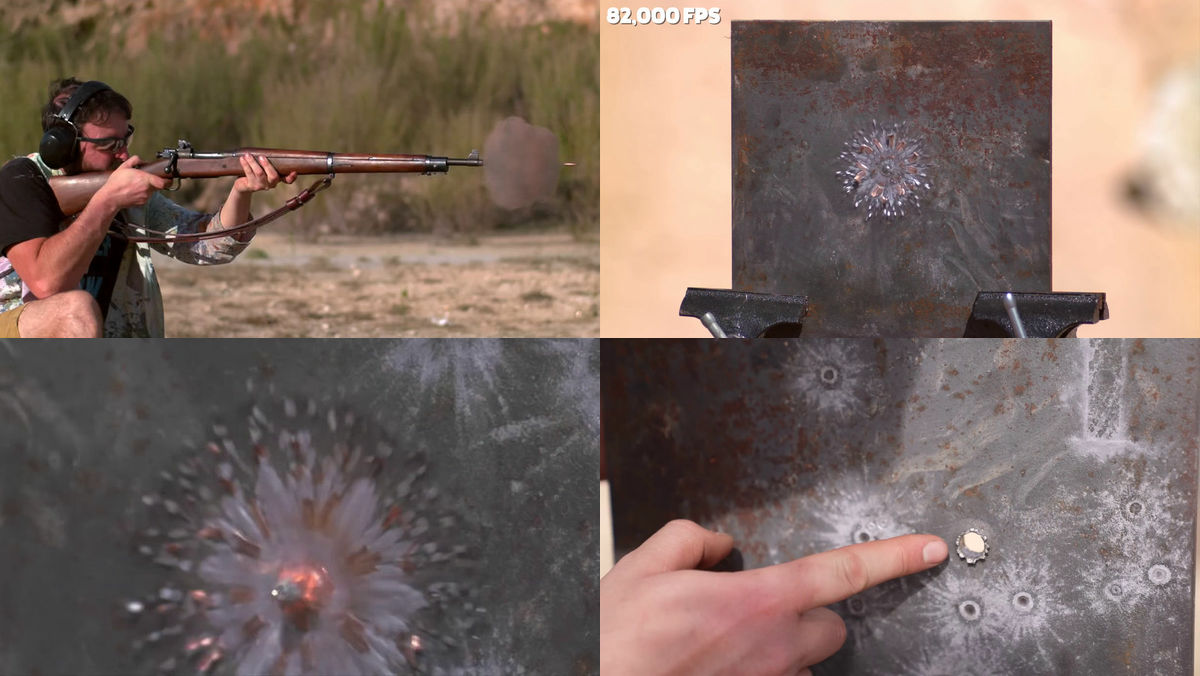The image consists of four rectangular photographs arranged in a grid, depicting a sequence of events involving a man shooting a rifle at a metal target. In the top left photograph, a man is seen firing an M1 Garand bolt-action rifle, characterized by a burst of smoke and a visible bullet exiting the barrel. He is wearing black protective ear covers, sunglasses, a camouflage jacket over his left shoulder, a short-sleeved black shirt, and khaki shorts, crouched down in a firing position.

The top right photograph shows the bullet impacting a steel plate, creating a radial pattern as it spreads out upon hitting the target. Notably, the corner of this photograph displays the label "82,000 frames per second," indicating the high-speed nature of the shot.

In the bottom left photograph, a close-up captures the exact moment the bullet strikes the metal plate, highlighting the radial splatter of bullet fragments and a slightly glowing area, suggesting the intense heat generated by the impact.

The bottom right photograph focuses on the back of the metal plate, revealing a large hole where the bullet penetrated through. A hand points to this hole, which is about the size of a dime, emphasizing the bullet's successful passage through the thick steel.

Together, these images provide a detailed, step-by-step visual analysis of the bullet's journey from the rifle to its point of exit through the metal target.